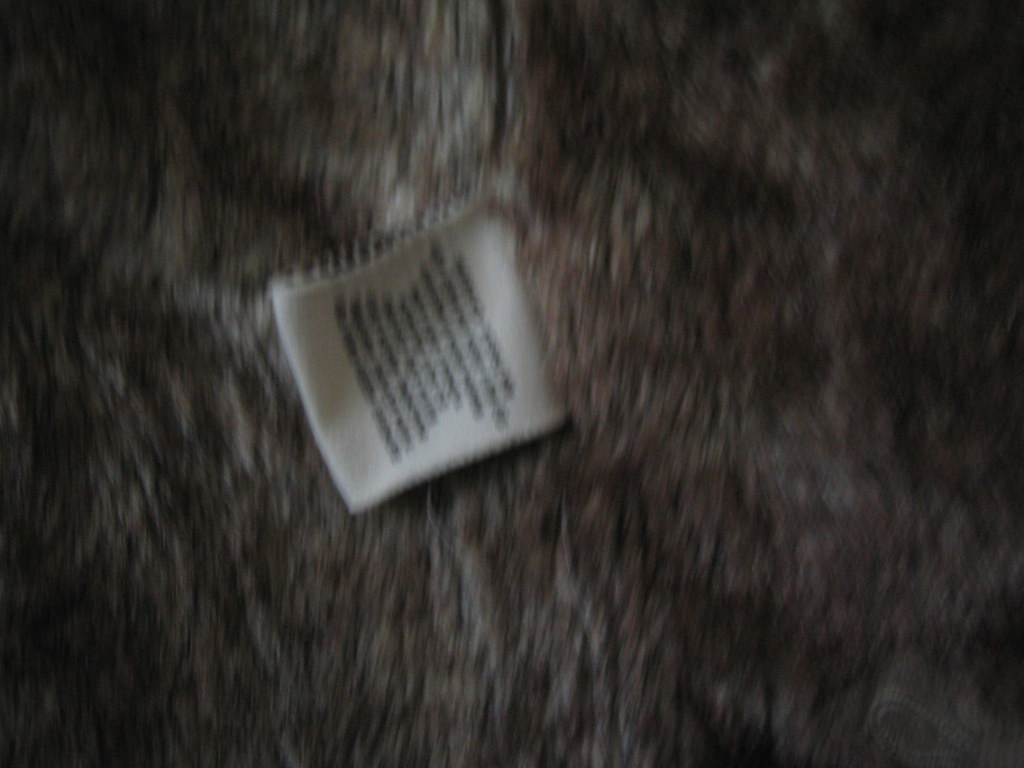The image depicts a close-up view of the interior tag on a garment, possibly a coat, sweater, hat, or any clothing item featuring a fur-like lining. The main focus is a small, white tag positioned in the center of the screen, folded over to the left, adorned with rows of black text that are too blurry to decipher. Surrounding the tag is a fur-like material, dark brown on the edges and lightening towards the center, suggesting a plush, possibly faux fur, polyester lining typical of winter garments. The overall appearance hints at a comfortable, warm material commonly used for linings to provide extra insulation. The setting and details of the tag strongly suggest it contains standard care instructions and material information.